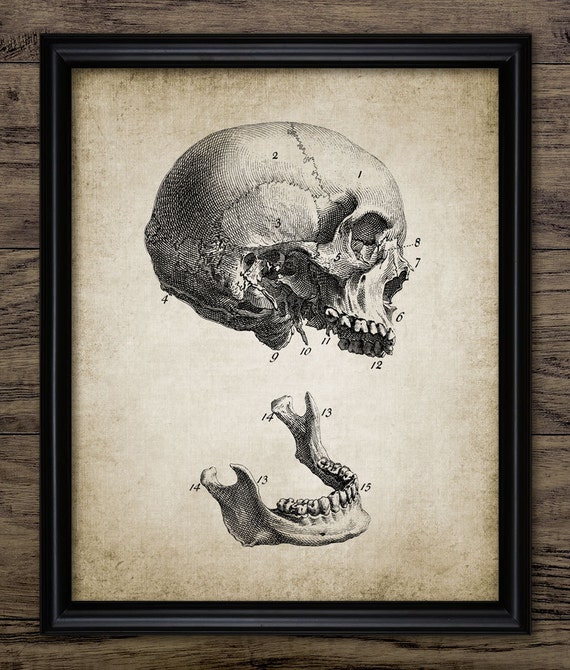A beautifully detailed lithograph of a human skull rests within a dark brown and light brown framed border atop a grayish wood-patterned table, where the striations in the wood are visible. The skull illustration is meticulously crafted with black lines and lighter shading, making the anatomical features discernible and precise. The image is oriented towards the right and displayed on a light brownish-white paper that fades to a darker shade towards the edges. The skull is separated into two sections: the upper part includes the eyes, nose, and upper teeth, while the lower jaw is detached and positioned below, showing the teeth and a ridge at the bottom of the skull. Numbers are carefully placed on various parts, including the teeth, eye sockets, and other bones of the head, with the forehead marked as number 1, and the jaw showing numbers 13, 14, and 15. Enclosed in a second black and shiny inner frame, this intricate anatomical illustration is a valuable resource for an anatomy class.